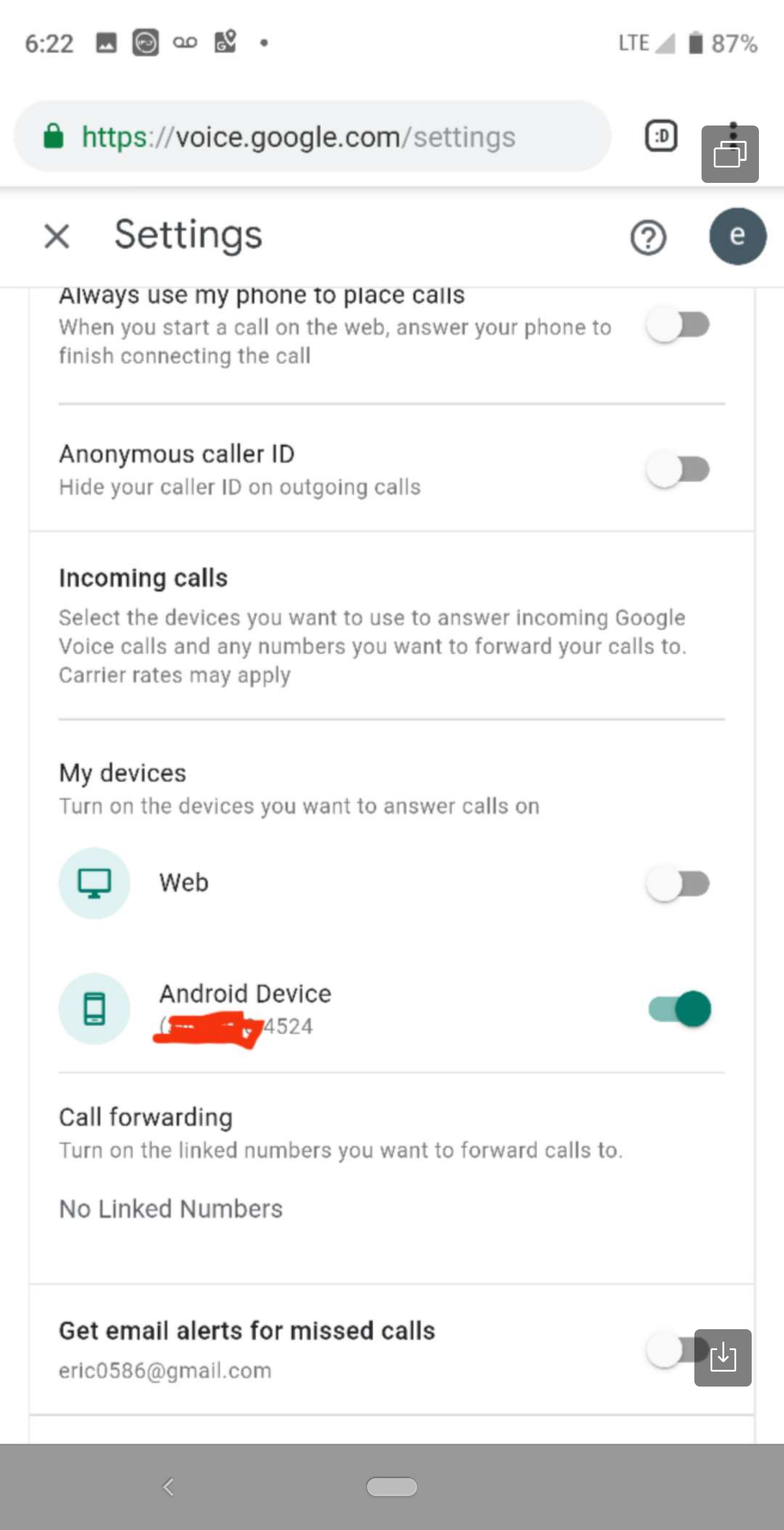A phone screenshot taken at 6:22 with an 87% battery level displays the "Google Voice Settings" page. The address bar reads "https://voice.google.com/settings". The page includes the following settings: 

1. "Always use my phone to place calls": Accompanied by a description stating, "When you start a call on the web, answer your phone to finish connecting the call." This feature's toggle bar is turned off.
   
2. "Anonymous caller ID": The description explains, "Hide your caller ID on outgoing calls." This toggle is also switched off.

3. "Incoming calls": The description advises users to, "Select the devices you want to use to answer incoming Google Voice calls, and any numbers you want to forward your calls to. Carrier rates may apply." Below a gray separator line, the section titled "My devices" appears.

- "Web": Turn on the device you want to answer calls on; the toggle bar for web is off.
- "Android device": This toggle bar is on, facilitating call answering on the Android device.

This comprehensive capture provides a detailed view of the user's current settings within the Google Voice platform.